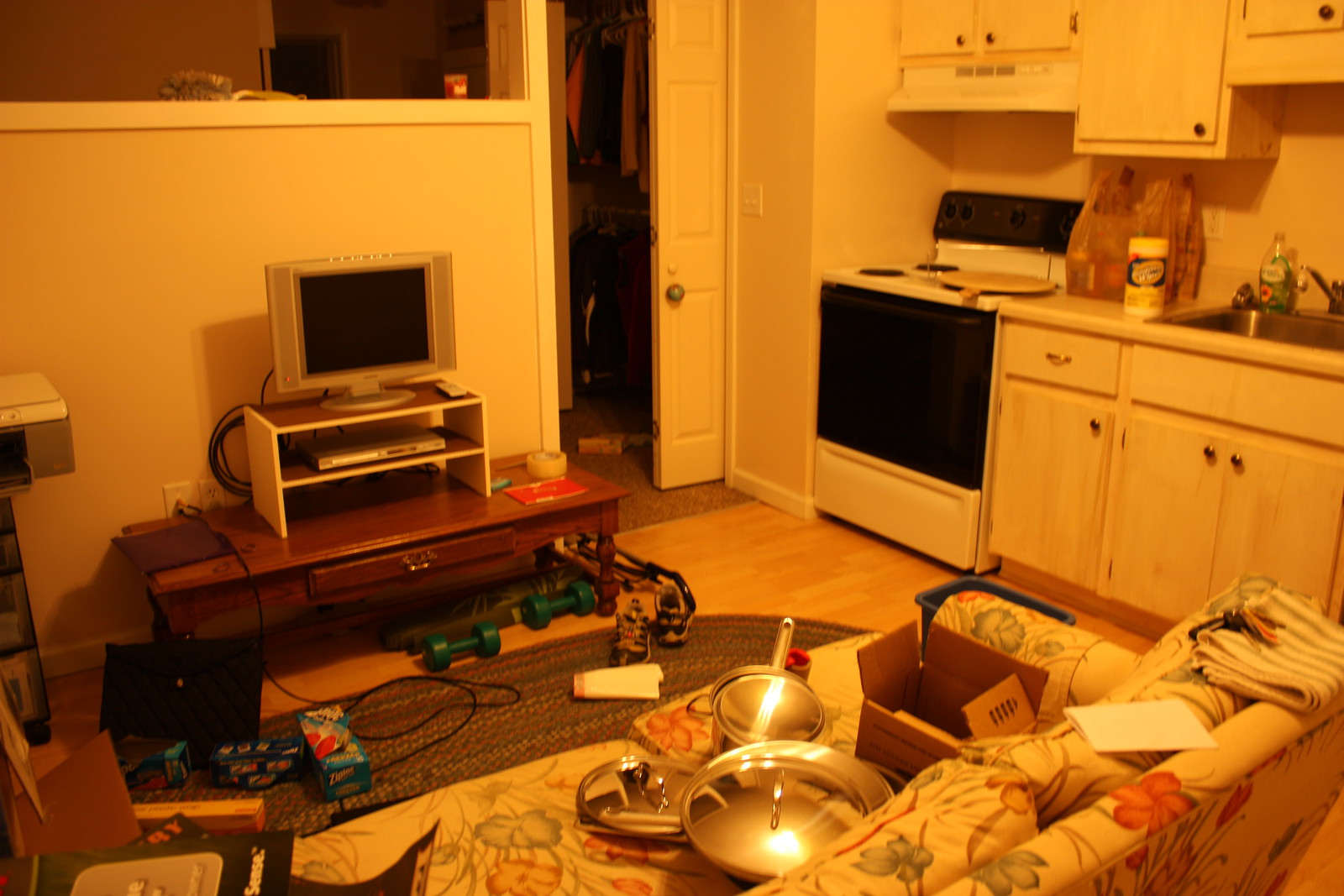This image captures an open floor plan living space, with the kitchen situated on the right side. The kitchen features white cabinets with metal handles, a white stove with a black door and range top, and a silver sink basin paired with a matching faucet. An assortment of items is visible on the countertop, including a clear bottle filled with green liquid—likely soap—and a canister with a white label adorned with a large blue section, presumably a cleaner.

Adjacent to the kitchen, toward the bottom left of the image, a white couch with a delicate floral pattern in shades of red, green, and possibly blue can be seen. The image has a yellow tint, making the colors slightly ambiguous. This couch is part of a cozy living area that also includes a small flat-screen TV flanked by speakers, standing on a light-colored entertainment stand. This setup rests on a wooden coffee table, complete with a brown throw rug draped over a light-colored wooden floor.

The overall ambiance of the space is warm and inviting, demonstrating a harmonious blend of functional kitchen area and comfortable living quarters.